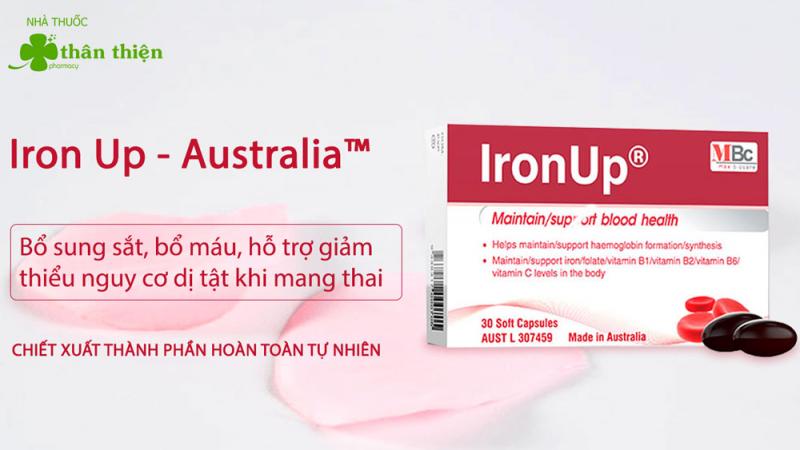The image showcases an advertisement for a product called Iron Up by Iron Up Australia. The background is light pink. On the bottom left, there is a green four-leaf clover emblem, with the accompanying text "N-H-A-T-H-U-O-C" in green and "Than Thien" to the right of the clover. Below this, in red text, it says "Iron Up – Australia™" followed by phrases in a red rectangular box that appear to be in Vietnamese: "Bo Sang Sat Bo Mau Ho Tro Jam Teun Gui Ko Di Tat Khi Mang Thai" and "Chet Sat Tan Than Hon Ton Thu Nien."

On the right side of the image, the main focus is a rectangular package box of the supplement Iron Up. The top of the package features the name "Iron Up" against a green rectangular section. Adjacent to this, in a smaller white rectangle, the text reads "NBC." Below this, it states "Maintain Support Blood Health" with additional descriptive text underneath. The package illustration includes three red capsules, and prominently at the bottom, it indicates "30 Soft Capsules made in Australia." In front of the package, there are two actual capsules shown, differing in color from the ones on the box—they are dark purple to black.

Overall, the advertisement effectively highlights the product's branding, association with blood health, and the distinction between the depicted red capsules and the actual dark capsules displayed.